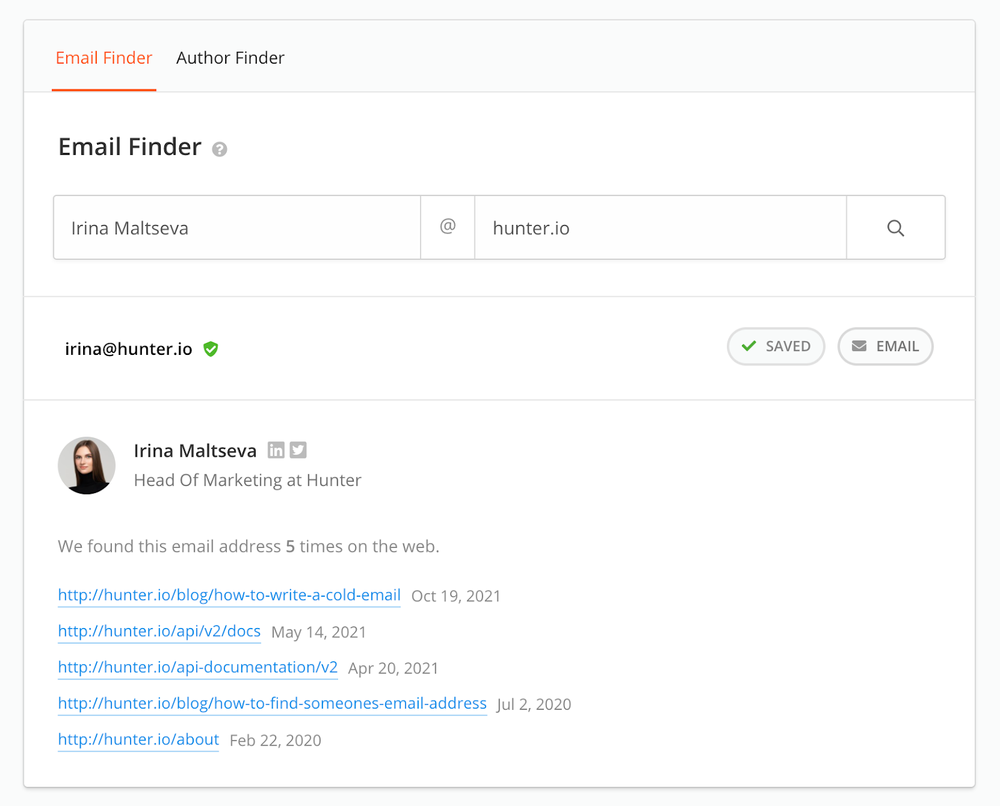On an off-white background with a gray border, this detailed email finder interface is presented. In the upper left corner, "Email Finder" is underlined in red, adjacent to "Author Finder" in black text. Below this, in black, white-spaced text, "Email Finder" appears beside a gray circle featuring a white question mark.

Following this, a series of labeled boxes offer user details:
- The first gray box reads, "Irina Matseva, M-A-L-T-S-E-V-A," followed by an at-symbol.
- The next box displays "Hunter.io," accompanied by a search icon.

A thin green line separates these elements from the email information. Below the line, in black text, "Irina at Hunter.io" is displayed beside a green shield icon with a white check mark. Two gray ovals appear beneath this:
- The first gray oval contains a green check mark with the text "Save" in gray.
- The second gray oval, marked with a gray envelope, reads "EMAIL" in capital letters.

A secondary thin green line traverses the interface beneath the ovals. To the right, there's a gray-toned profile picture of Irina Matseva, showcasing her brown hair, black turtleneck, and a warm smile. The caption describes Irina as the "Head of Marketing at Hunter."

The interface also indicates that Irina's email address was found five times on the web, with each instance highlighted in blue. The sources are listed chronologically:
1. Blog, "How to Write a Code Email," October 19, 2021
2. API V2 Docs, May 14, 2021
3. API-Documentation-V2, April 20, 2021
4. Blog, "How to Find Someone's Email Address," July 20, 2020
5. About, February 22, 2020